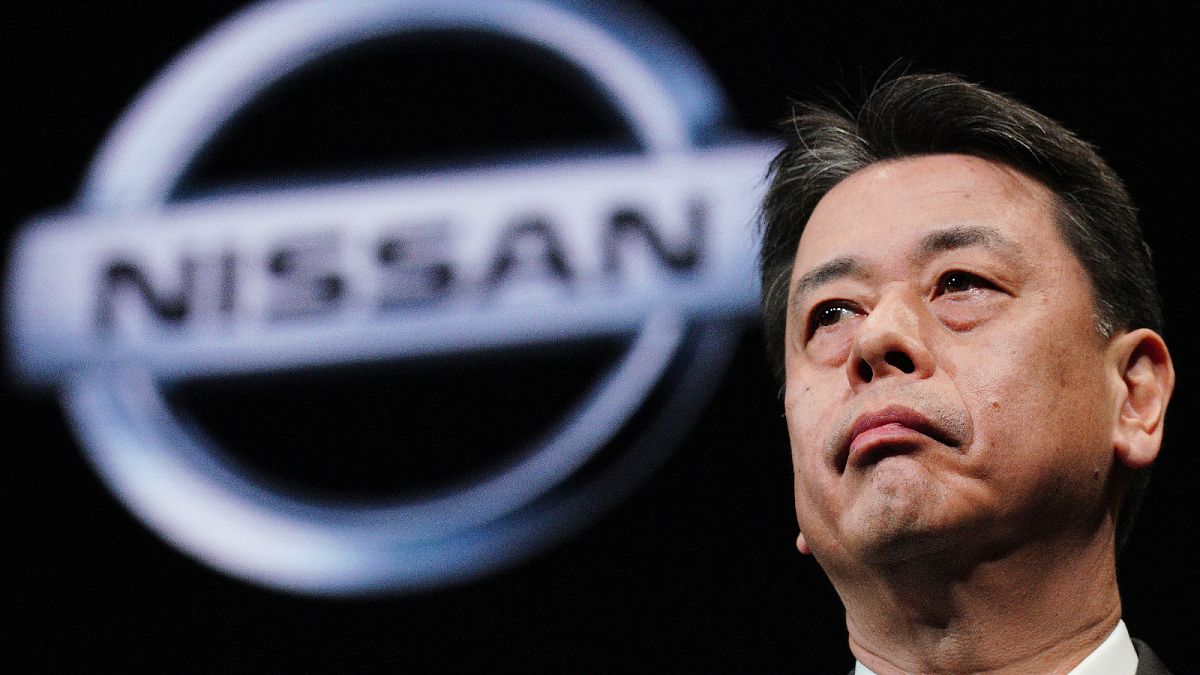The photograph captures a man of Asian descent, likely in his 50s or 60s, with black hair interspersed with gray strands, cut short and parted in the middle. He has notable crescent-shaped eyes and a clean-shaven face marked by a somber, grim expression, suggesting unhappiness or concern. Dressed in a suit with a collared white shirt, he stands against a black background. Behind him, slightly out of focus, is a large silver Nissan logo composed of a circle intersected by a rectangular banner bearing the company's name in black letters. The man appears to be addressing a crowd, possibly as a leader or executive of the Nissan Corporation, amid a setting that hints at possibly disappointing news.